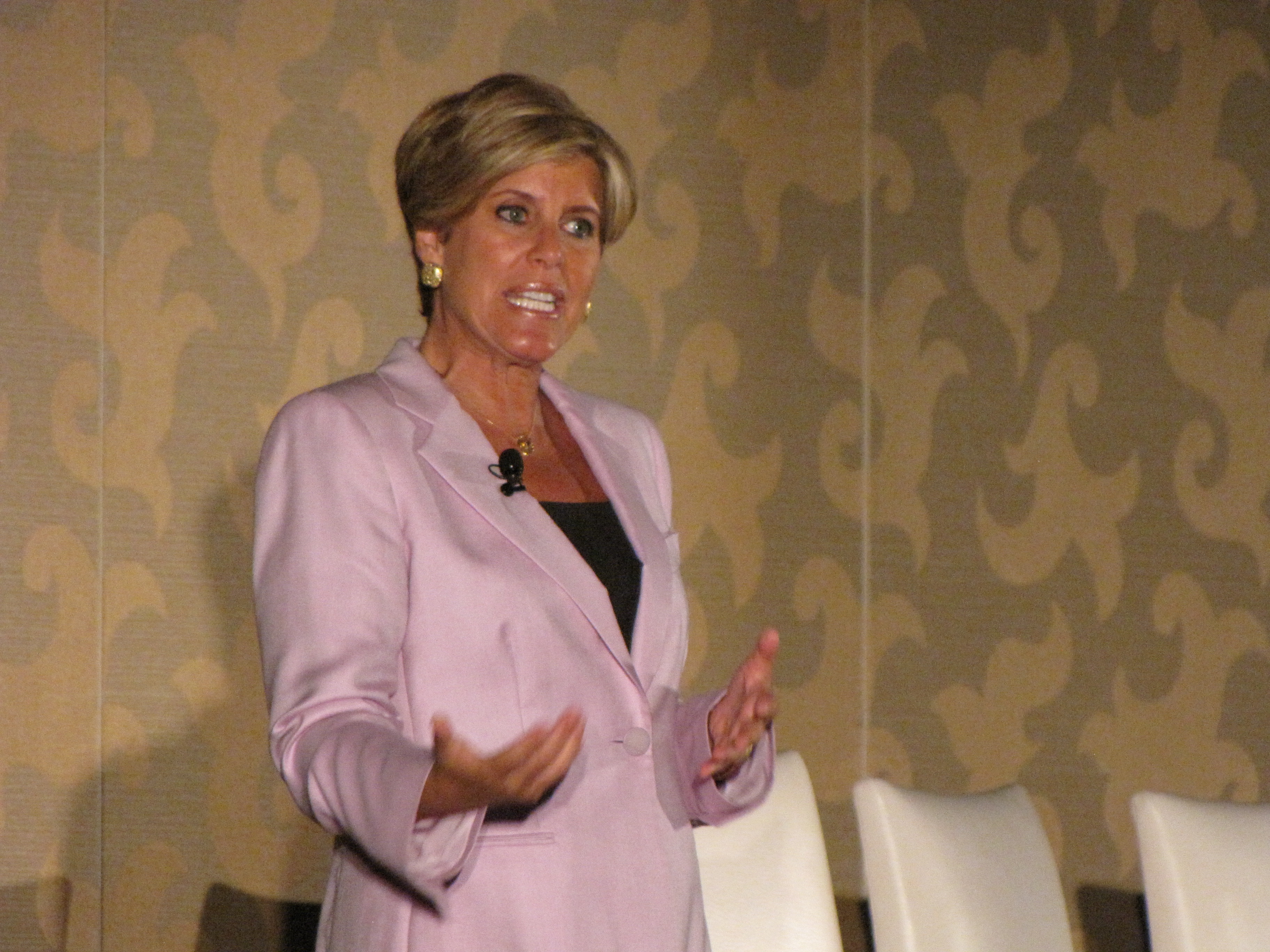The photograph captures a middle-aged woman, possibly Susie Orman, speaking, with her mouth open and mid-gesture, her palms facing upward. She is viewed from the waist up, facing towards the right side of the image and looking at something out of frame. She wears a light pink business coat with a single clasped pink button, featuring a pocket near the bottom. Attached to the lapel is a small black microphone. Underneath the coat, she has on a low-cut black top, accessorized with a gold chain necklace that features a large oval pendant. She also sports large circular gold earrings. Her hair is short, styled in a fashionable, slightly voluminous manner, and is a dirty blonde color. The background has a golden-brown hue with light gold curly designs, and towards the bottom right of the image are several empty white cushioned chairs.